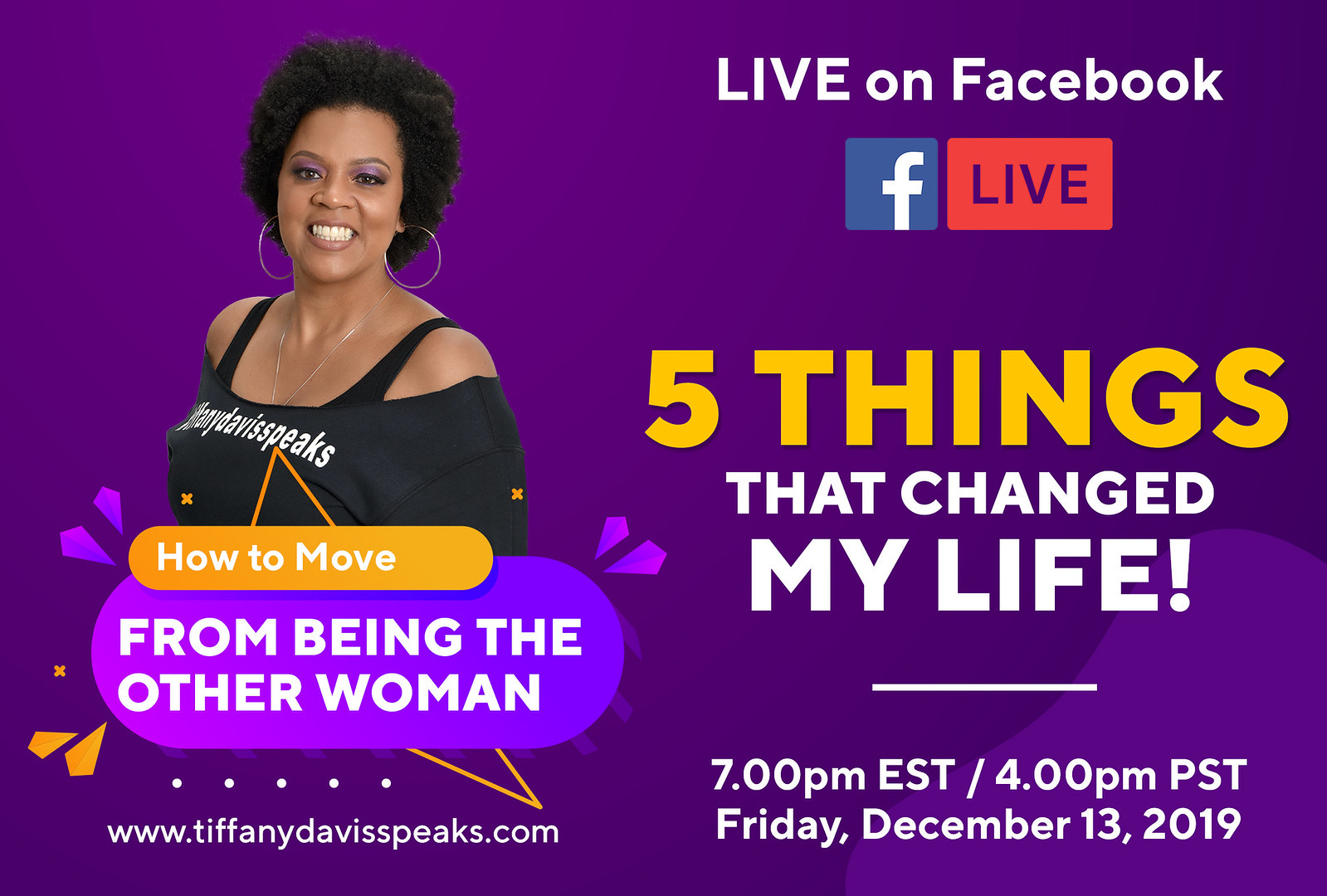This advertisement, likely designed for online promotion, is formatted as a wide rectangle with a purple background. 

On the left side, a smiling black woman with curly hair is prominently featured. She wears large hoop earrings, purple eyeliner, and a black top that reveals part of her bra. The top has partial text visible, likely including "speaks." 

Below her image, the text reads, "How to Move from Being the Other Woman." The advertisement announces a live session on Facebook, featuring the Facebook logo and the word "Live." In large yellow letters, it highlights "Five Things" and in slightly smaller white text, "that Changed My Life!" 

The event details are clearly stated: 7 PM Eastern / 4 PM Pacific on Friday, December 13, 2019. At the bottom left, the web address "www.tiffanydavisspeaks.com" is provided, directing viewers for more information. This session appears to offer insights and personal experiences about transitioning from being 'the other woman' in a relationship.